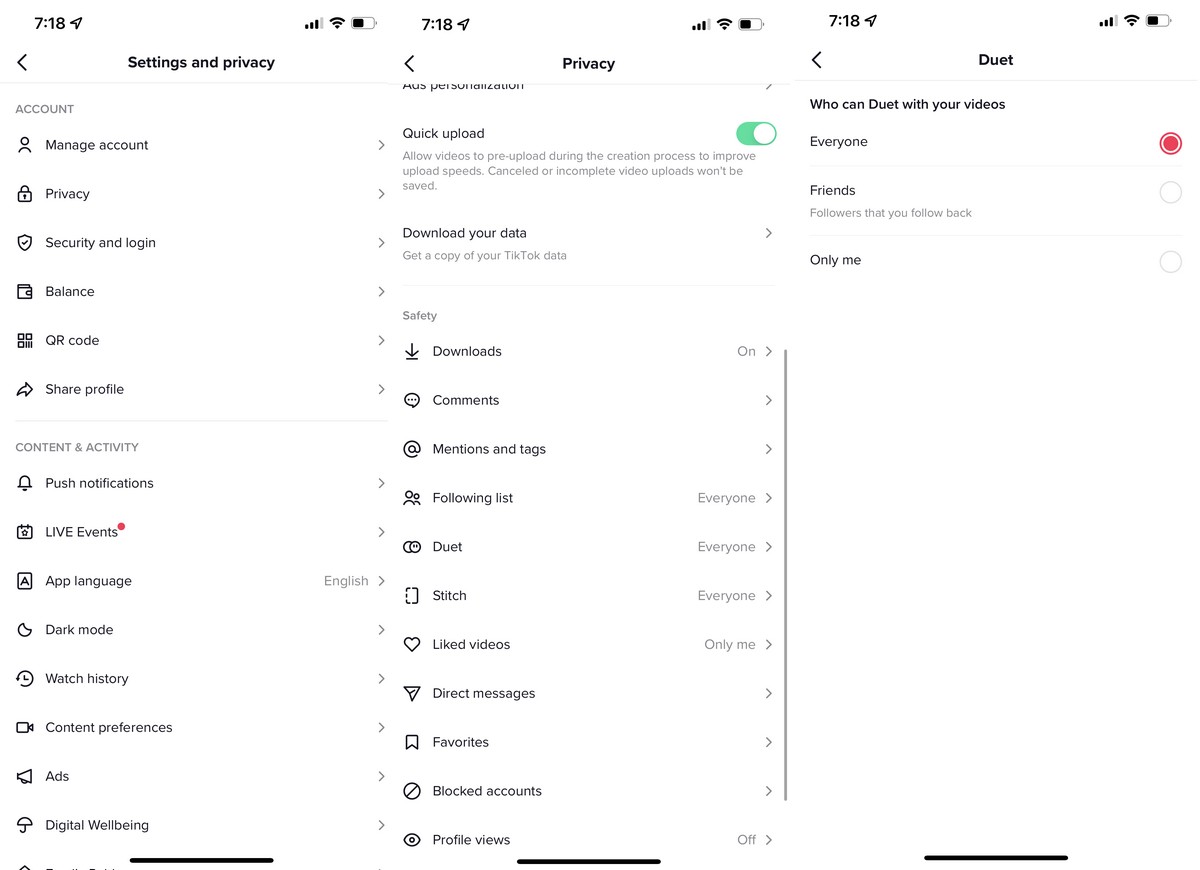Here are three detailed, cleaned-up captions for each screenshot described:

1. **Screenshot 1: Settings and Privacy Overview** 
   The screenshot features the 'Settings and Privacy' section of a mobile phone interface, categorized into multiple sub-sections. Under 'Account,' users can manage settings such as 'Account Management,' 'Privacy,' 'Security and Login,' 'Balance,' 'QR Code,' and 'Share Profile.' The white background prominently presents the clearly labeled options, and the time noted on the top left corner is 7:18.

2. **Screenshot 2: Content, Activity, and Safety Settings**
   Displaying the 'Content and Activity' portion under the 'Settings and Privacy' menu, this screenshot highlights a 'Live Events' option marked with a red notification dot. Additionally, the 'Privacy' section is visible, where 'Quick Upload' is toggled green. Users are also provided with the option to 'Download Your Data' listed below 'Quick Upload.' In the 'Safety' section, various settings include 'Download,' which is enabled, 'Following List' set to 'Everyone,' 'Duet' and 'Stitch' both set to 'Everyone,' 'Liked Videos' set to 'Only Me,' and 'Profile Views' set to 'Off.' The screencap maintains a clear white background, with the time stamp reading 7:18 on the top left corner.

3. **Screenshot 3: Duet Permissions**
   This screenshot details the 'Duet' settings under the 'Privacy and Safety' section. The primary query 'Who can duet with your videos?' is shown, with 'Everyone' option toggled in red. Alternative options like 'Friends,' 'Followers that you follow back,' and 'Only Me' have no active toggles. Maintaining consistency, the background remains white, and the time stamped at the upper left is 7:18.

Each screenshot effectively captures detailed configuration settings within a clean, white interface, providing essential information at a glance along with a consistent time display.